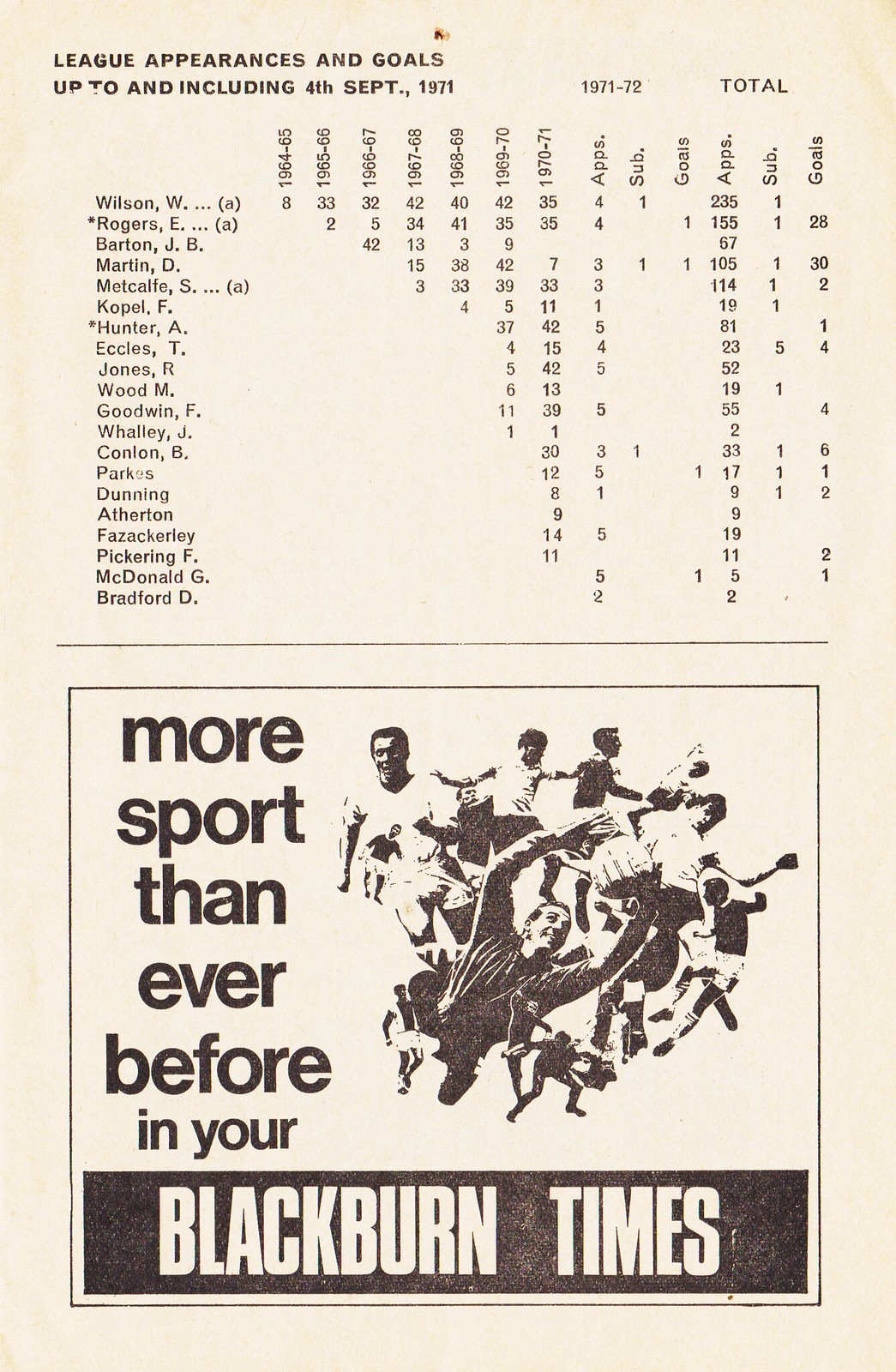This photograph showcases a rectangular, cream-colored poster that appears to be a page from an old magazine or program. The top left corner features brownish text reading, "League Appearances and Goals up to and including 4th September 1971." A detailed list of player names is organized along the y-axis, including individuals such as Wilson W., Rogers E., Barton J.B., and more, while the x-axis chronicles the years from 1964 to 1971, with sections for appearances (apps), substitute appearances (sub), and goals. 

Below this list, a black and white drawing depicts players in various playing positions. Adjacent to this illustration, a caption reads, "More sport than ever before in your Blackburn Times," with "Blackburn Times" highlighted in white print set against a black footer at the bottom. The overall design and text placement suggest that this document serves as a historical record of player statistics, and its aged, tan hues hint at its vintage origin.